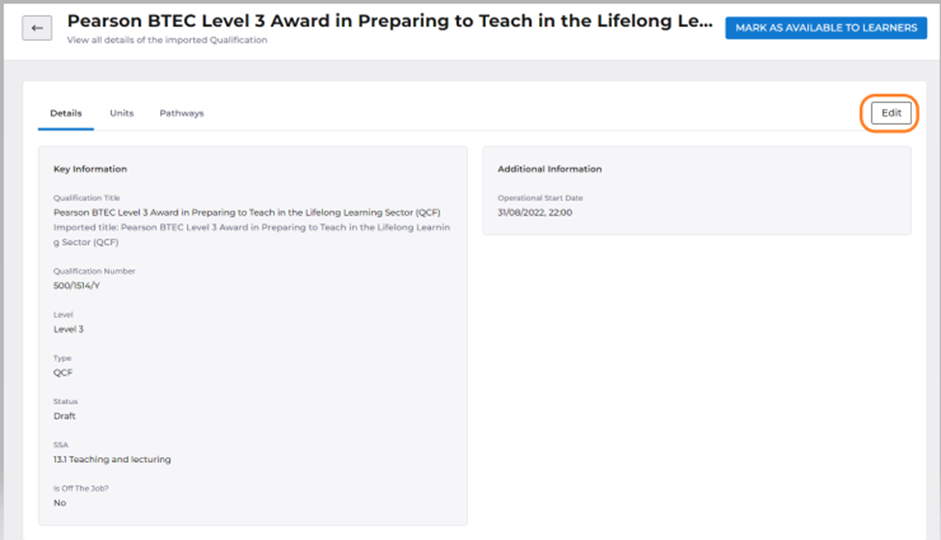This landscape-oriented screenshot appears to capture a user interface of an educational or coding application. The interface features a thicker gray border on the left and top sides, a thin gray border on the right, and no bottom border.

At the top of the interface, there is a long, white rectangular box separated by a thin gray line. The header within this box reads "Pearson BTEC Level 3 Award and Preparing to Teach in a Lifelong LE..." but the text is slightly cut off. To the left of this header, a gray rectangular box with a left-pointing arrow and the text "View All Details of Imported Qualification" is visible. In the upper right corner, a long, narrow blue box with white font displays the text "Mark as Available to Learners."

Beneath this section, the area transitions to a gray background featuring a long, white rectangular box. The box has a thin gray border across the top, forming a header with three options on the left: "Details," "Units," and "Pathways." The "Details" option is in bold with a blue underline, indicating it is currently selected. To the right of these options, an "Edit" button is present, which is rectangular in black with a white background and encircled by an orange oval.

Below this header, two gray box columns are positioned. The first column, labeled "Key Information," lists several pieces of information, while the smaller second column is labeled "Additional Information."